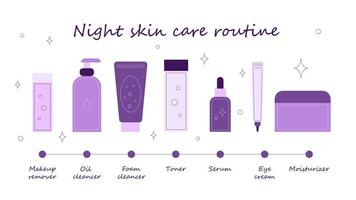This digital illustration presents a detailed example of a night skincare routine. The background is white, while almost every other element is in various shades of purple, giving the design a cohesive and soothing aesthetic. The top of the illustration features the title "Night Skincare Routine" in a blackish, somewhat cursive font. Below the title, the routine is visually laid out from left to right, beginning with makeup remover and followed by oil cleanser, foam cleanser, toner, serum, eye cream, and moisturizer. Each step is accompanied by a minimalist, flat design illustration of the corresponding product, all depicted in shades of purple. Tiny stars, white-centered with purple outlines, are interspersed throughout the image, adding whimsical detail. This clear and aesthetically pleasing diagram effectively showcases a complete night skincare regimen.